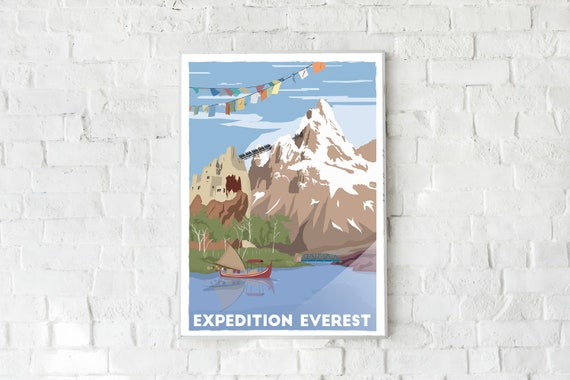The image depicts a rectangular poster with a white inner border and a thin metal frame, mounted on a white painted brick wall. This commercial-style photo, often used for online listings, catalogs, or websites, showcases a cartoon graphic of a vast, snow-covered mountain range. In the foreground, a river with an Asian-style curved boat streams through a lush green area dotted with white trees. To the right of the mountain, temples and buildings are visible. The sky above the scene transitions between various blue hues, adding depth to the image. Colorful square flags are strung across the upper left corner of the poster, adding a festive touch. At the bottom, white text reads "Expedition Everest," underscoring the adventurous theme of the artwork.